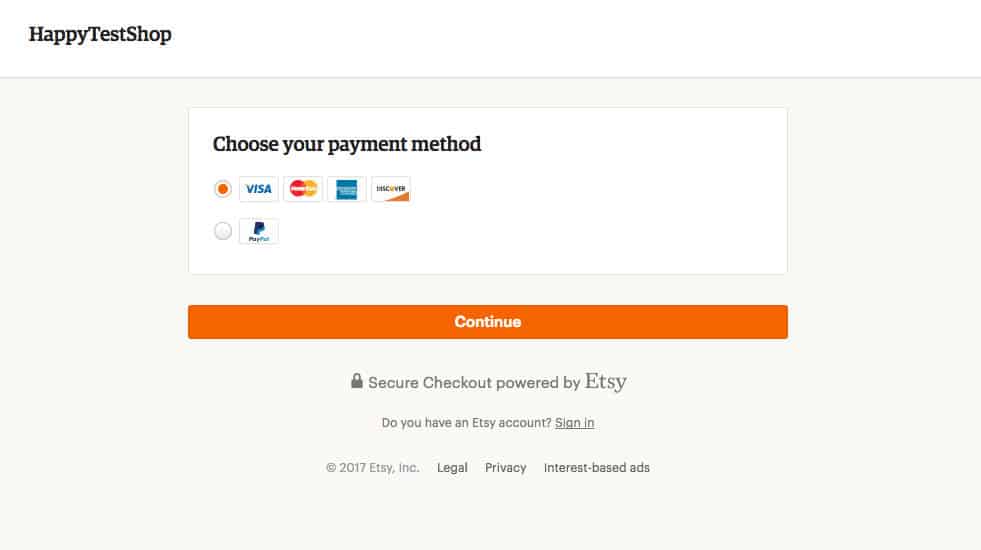This image depicts a webpage interface for an online shop named "Happy Test Shop." At the top left corner, the shop's name is prominently displayed. Below, the page instructs users to choose their payment method. The first payment option is via card, with supported card types including Visa, MasterCard, and Discover. The second payment option available is PayPal. Towards the bottom of the page, there is a "Continue" button, emphasizing a secure checkout experience powered by Etsy. For existing Etsy users, there's a prompt to sign in. The footer of the page contains legal and privacy information, stating copyrights held by Etsy, Inc. for the year 2017, and mentions about interest-based ads. The page features a color palette that includes black, orange, blue, red, white, and gray.